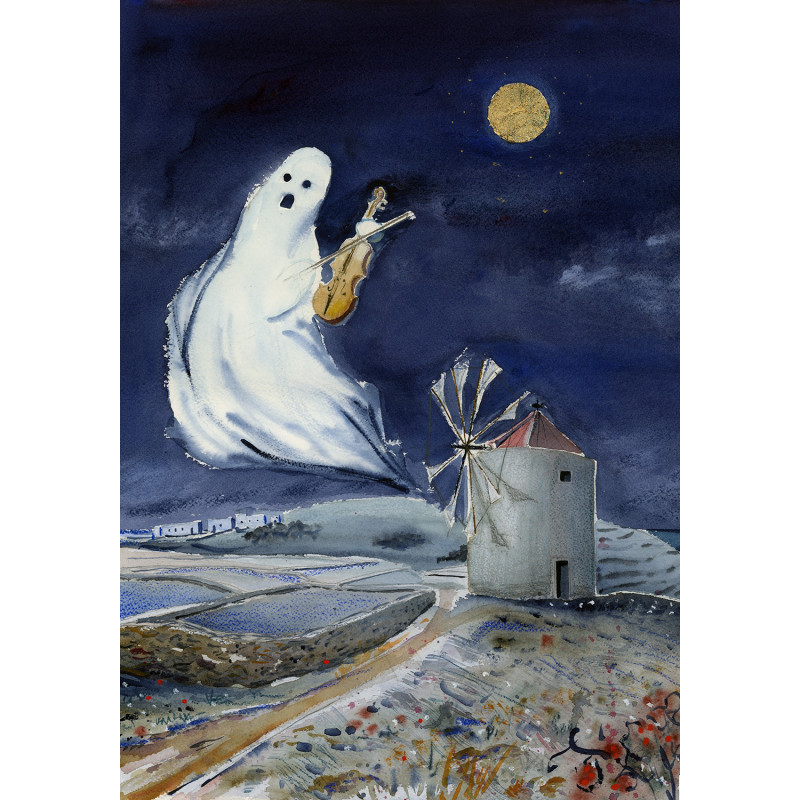This detailed painting depicts a ghostly figure floating above a wintry landscape at night. The spectral apparition, significantly larger than its surroundings, hovers on the left side, grasping a violin and its bow in its ethereal paw-like hand. The ghost appears to be emerging from a white windmill with a tall reddish roof located at the center right of the composition. The dark blue night sky is illuminated by a bright yellow moon in the upper right corner, accompanied by wispy gray clouds. Below, a dirt road stretches from the lower left corner towards the windmill and seems to vanish into the distance, implying a path that leads to a small town made up of several white buildings on the far left. The ground, scattered with patches of blue and white that suggest snow, features occasional red and brown spots, indicating plants breaking through the frost. A cement fence or barrier parallels the road, adding to the sense of structure in this cold, surreal winter night scene.